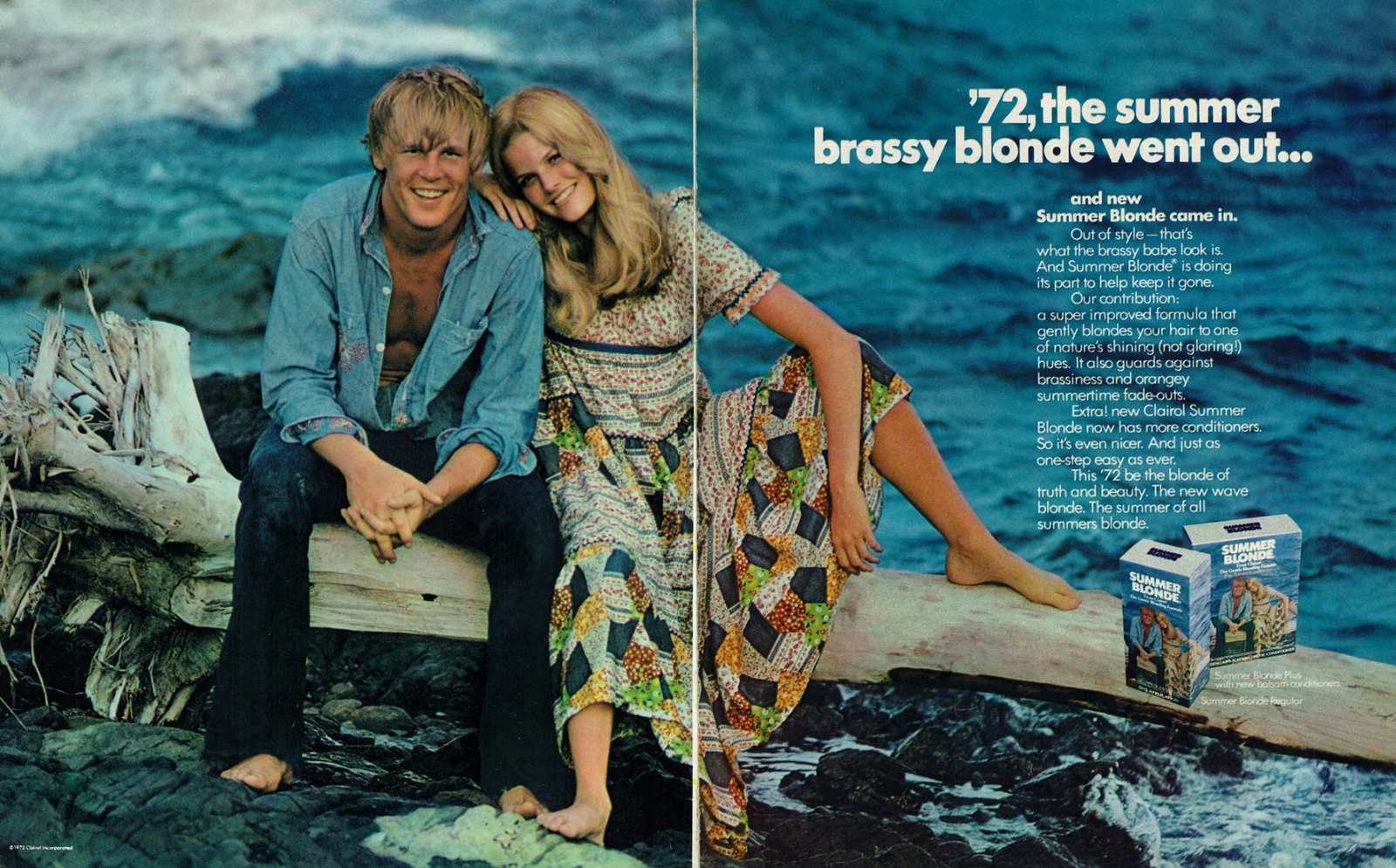The magazine features a stunning double-page spread that captures a young couple at a beach. The left page primarily showcases the young man and woman sitting barefoot on a large piece of driftwood, while the right page has the woman slightly extending into it. With the blue ocean and waves forming a serene backdrop in the upper left corner, the scene is both picturesque and inviting. The man, sporting a tousled look, is dressed in an unbuttoned denim shirt over a t-shirt, paired with blue jeans that flare out at the bottom. His blonde hair falls over his ears and just above his eyebrows, and he is flashing a broad smile. Beside him, the woman radiates joy with her long blonde hair cascading over her shoulders. She is wearing a handcrafted-looking, multicolored dress adorned with patterns resembling squares and patch-like designs in various hues of blue, orange, and green.

At the top right of the spread, a bold text reads, "72, the summer brassy blonde went out" with smaller text beneath it stating, "and new summer blonde came in." Below this headline, additional text describes the new hair dye product, emphasizing its improved conditioning and ease of use. The advertisement is for Clairol's "Summer Blonde" hair dye, with two small product boxes pictured at the bottom of the spread, reinforcing the magazine's promotional intent. The couple's relaxed, happy demeanor perfectly encapsulates the carefree spirit of a summer makeover.